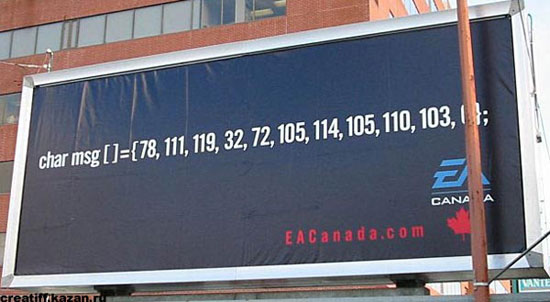**Descriptive Caption:**

An outdoor billboard prominently displays a textual message in red and black fonts. The message reads: "car message Boxes" followed by an enigmatic sequence of numbers and symbols: "[7811119 32 72 105 114 105 110 103 0]". Below this cryptic text, the words "EA Canada" are printed twice, along with a URL reading "EACanada.com." The backdrop of the billboard includes a brick building situated in the top left corner of the frame, partially obscured by the sign. On the right side of the billboard, a sturdy wooden post stands erect. Contributing to the Canadian theme, a red maple leaf, a symbol of Canada, is visibly located at the bottom right corner of the poster.